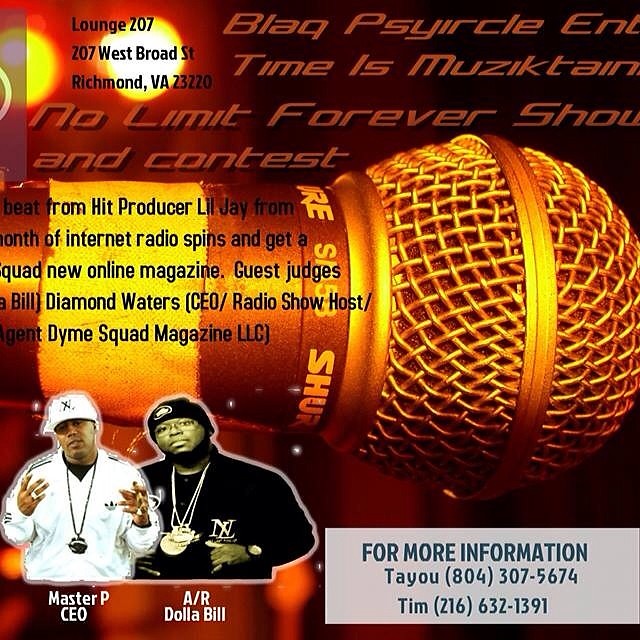This image is an advertisement for a music event or contest by Black Cycle Entertainment, set against a dark background with various colorful elements. At the center, there's a close-up illustration of a microphone, starting from the top right and stretching horizontally across the image. Above the microphone, the text mentions the event location: "Lounge 207, 207 West Broad Street, Richmond, Virginia, 23220." 

Prominently displayed across the shaft of the microphone are details about the event, though some text is cut off: "Beat from hit producer Lil Jay, from Month of Infinite Radio Spins, and Get a Quad New Online Magazine." Guest judges include Bill Diamond Waters, CEO and radio show host, along with others from Dime Squad Magazine, LLC. 

In the bottom left corner, there are images of two artists: Master P, wearing white, and AR Dollar Bill, wearing black, both adorned with necklaces. The bottom right corner features two gray rectangular banners providing contact information: "For more information, contact Taiyu at 804-307-5674 or Tim at 216-632-1391."

Overall, the flyer features a palette of gold, brown, white, black, gray, yellow, orange, red, and dark gray colors, giving it an eye-catching and vibrant appearance designed to attract attention to the event.